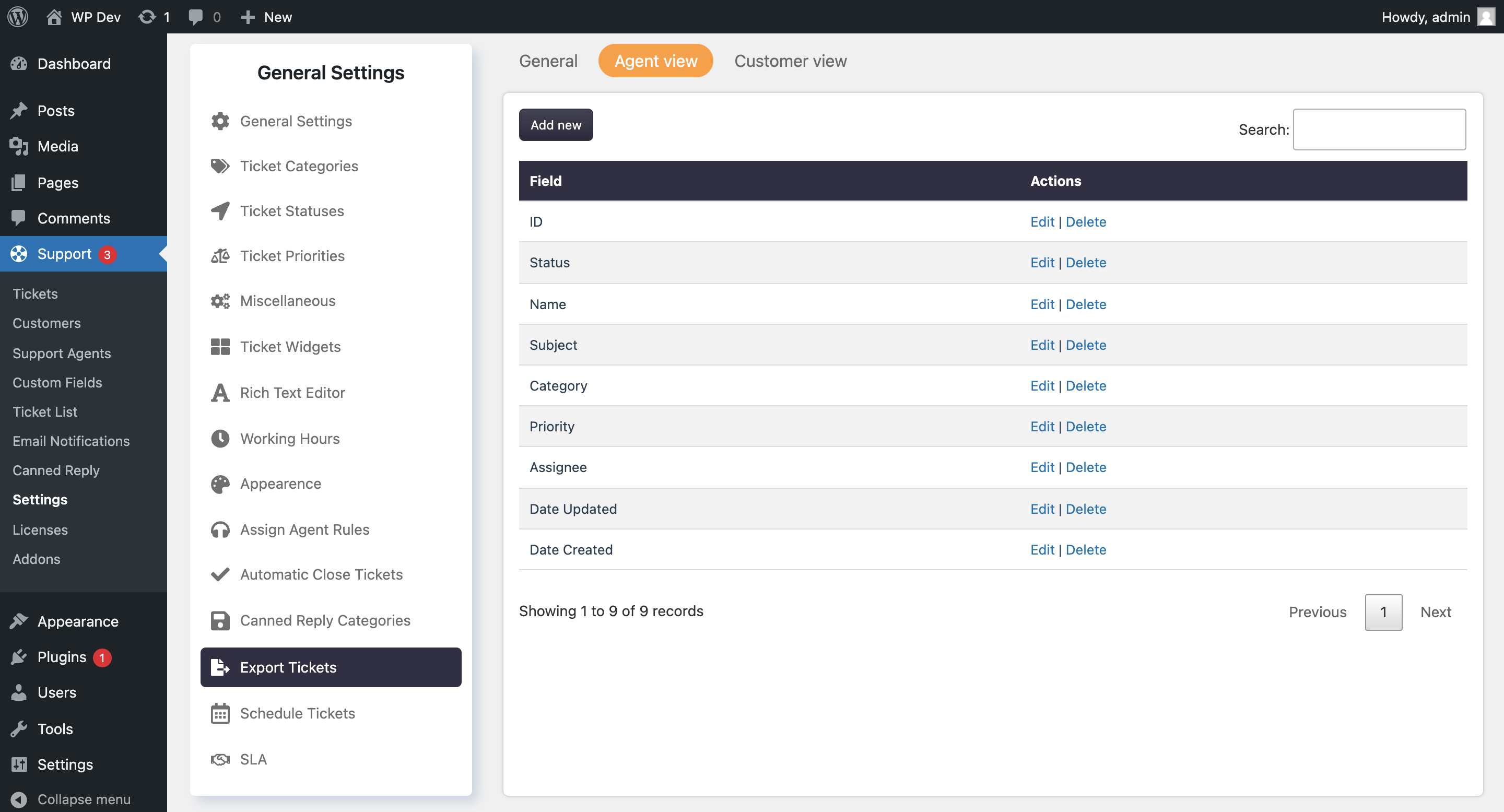In this image, we see a detailed screenshot of a settings menu within a WordPress admin dashboard, likely focusing on a customer support or ticketing system. Starting from the top, there is a black panel featuring the WordPress icon, followed by a notification bubble with the numbers "1" and "0", a chat icon, a "Plus New" button, and a "Howdy, admin" message positioned on the far right.

On the left side, a vertical black sidebar houses various navigation icons and categories. These include:

- Dashboard 
- Posts 
- Media 
- Pages 
- Comments 
- Support (highlighted in blue with three unread messages)
- Tickets
- Custom Fields
- Ticket List
- Email Notifications
- Canned Replies
- Settings
- License Add-ons
- Appearance
- Plugins
- Users 
- Tools 
- Settings 
- Compose Menu

Adjacent to "Support" is a small arrow pointing towards a larger white list area on the right, detailing multiple settings options such as:

- General Settings
- Ticket Categories
- Ticket Statuses
- Ticket Priorities
- Miscellaneous
- Ticket Widgets
- Rich Text Editor
- Working Hours
- Appearance
- Assigned Agent Rules
- Automatic Closed Tickets
- Canned Replies
- Categories (highlighted in black)
- Export Tickets
- Scheduled Tickets
- SLA

To the right of the vertical sidebar, there is text labeled "General," beneath which sits an orange rectangle labeled "Agent View" in white, and "Customer View." It appears the "Agent View" is currently selected.

Below this, a black rectangular button labeled "Add New" accompanies a search bar, followed by another black bar that reads "Fields" and "Actions." The area below displays rows of ticket data with blue "Edit" and "Delete" options for each action. The columns include:

- ID
- Status
- Name
- Subject
- Category
- Priority
- Assignee
- Date Updated
- Date Created

At the bottom of the list, it indicates "Showing 1 to 9 of 9 records," with navigation buttons on the bottom right reading "Previous" and "Next," where "1" is within a square box, likely indicating the current page.